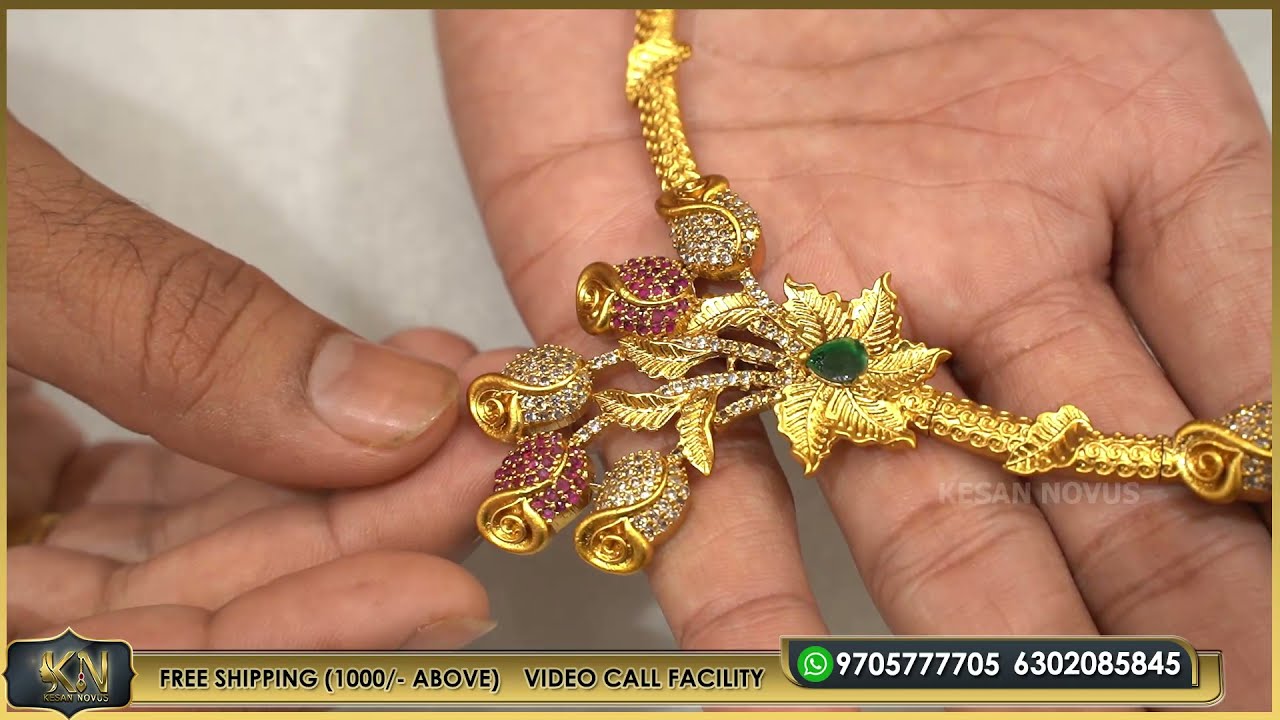The image showcases two hands against a black background, elegantly presenting a gold necklace adorned with floral and rose designs. The hand on the right side of the picture, with caramel-colored skin, gently holds the intricate jewelry, which features gold leaves, white stones along the stems, and vibrant red stones embedded in the roses. There's also a prominent green gem in the design, adding a striking contrast. The left hand delicately adjusts the rose heads, showcasing the piece from different angles. At the bottom of the image, a gold-bordered banner reads, "KESAN Novus." Below this, text advertises "Free shipping for 1000 and above" and mentions a "video call facility," alongside WhatsApp contact numbers 970-577-7705 and 630-208-5845, neatly displayed with the WhatsApp logo in white text.